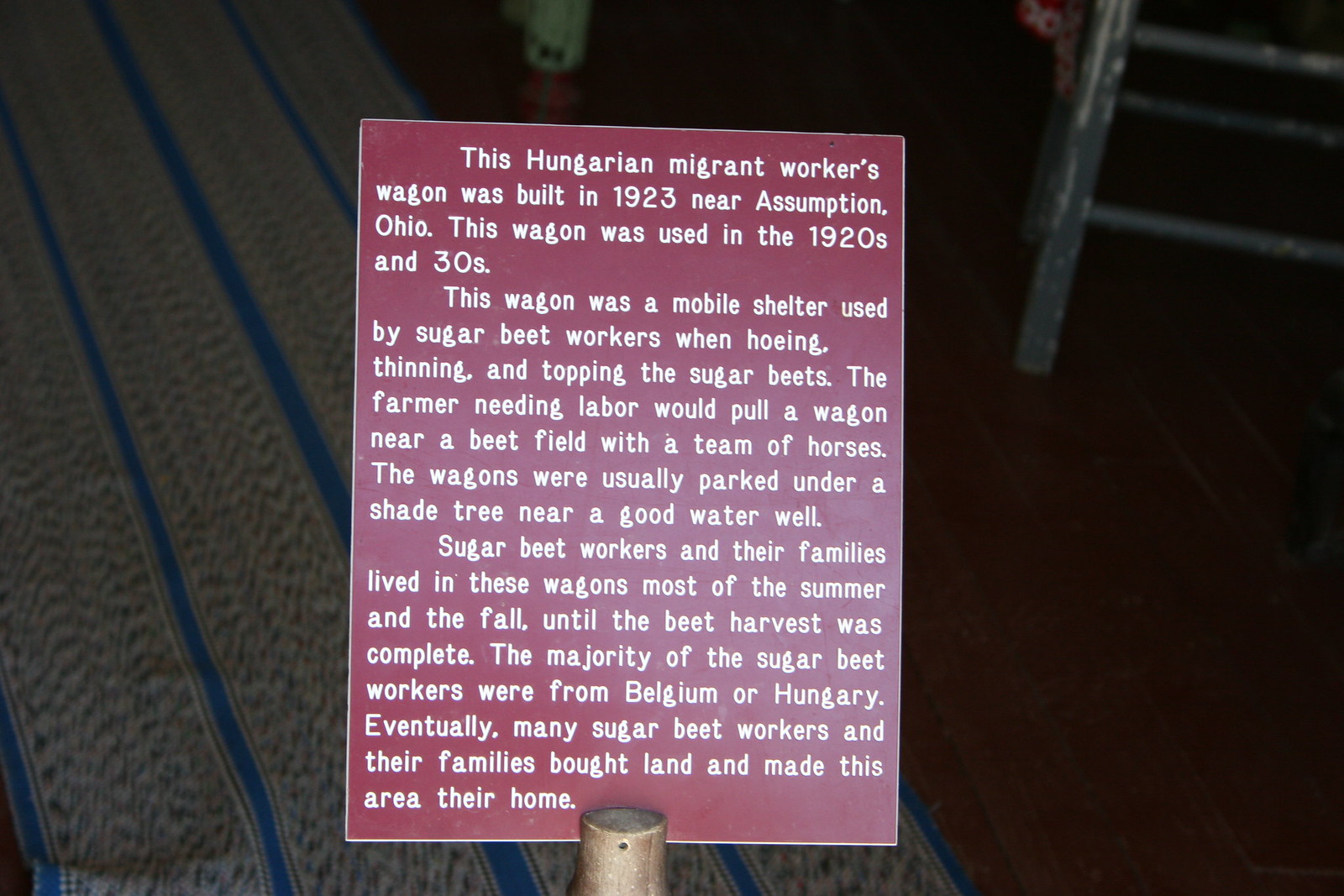The image displays a red information card with white text, describing a Hungarian migrant workers' wagon built in 1923 near Assumption, Ohio. This mobile shelter was used by sugar beet workers during the 1920s and 30s for hoeing, thinning, and topping sugar beets. Farmers would pull these wagons with a team of horses to beet fields, and they were typically parked under shade trees near a good water well. Sugar beet workers and their families lived in these wagons throughout most of the summer and fall until the beet harvest was completed. The majority of these workers were from Belgium and Hungary. Over time, many sugar beet workers and their families settled in the area, purchasing land and establishing permanent homes. The background includes a gray rug with blue stripes, wooden flooring, and the bottom of a stool or chair with worn-off paint, adding context to the scene.